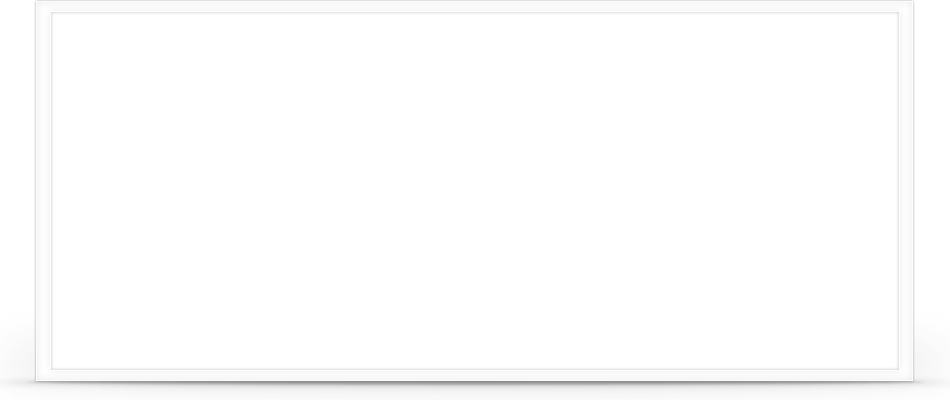A minimalist image depicting a horizontally elongated white rectangle, bordered by a slightly different shade of white, against a white background. The outer border is relatively thin in comparison to the size of the central rectangle, creating a subtle, almost invisible contrast. This composition focuses solely on the interplay of white tones and geometric simplicity, devoid of any additional elements or textural details.